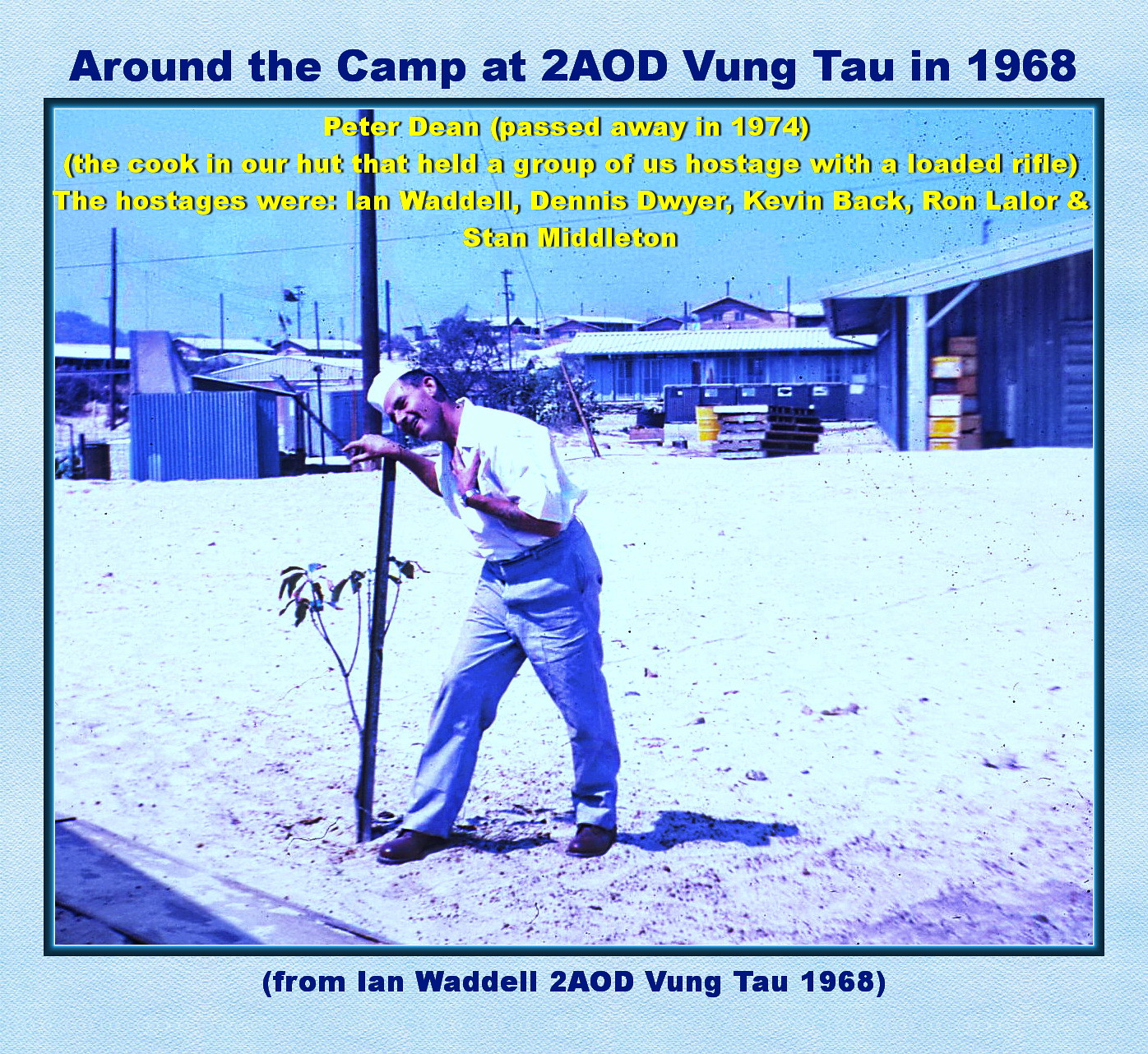This historic photograph, framed with a blue border, captures an image from 1968 at the 2AOD camp in Vung Tau, Vietnam. The central figure, identified as Peter Dean—a cook who later held his hutmates hostage with a loaded rifle—is leaning casually against a post or tree emerging from the sandy ground. Peter, who wears a sailor's cap, a white button-down shirt, gray pants, and brown shoes, looks contemplatively to the left. His legs are slightly apart, one arm resting on the post and the other clutched over his chest. The sandy foreground blends into a backdrop of wooden, single-story buildings with white roofs, alongside stacks of pallets. Yellow text overlays the image, providing poignant context: "Peter Dean passed away in 1974. The cook in our hut that held a group of us hostage with a loaded rifle. The hostages were Ian Waddell, Dennis Dwyer, Kevin Back, Ron Laylor, and Stan Middleton." The top border features the inscription, "Around the camp at 2AOD Vung Tau in 1968," while the bottom reads, "From Ian Waddell 2AOD Vung Tau 1968," both in blue text.